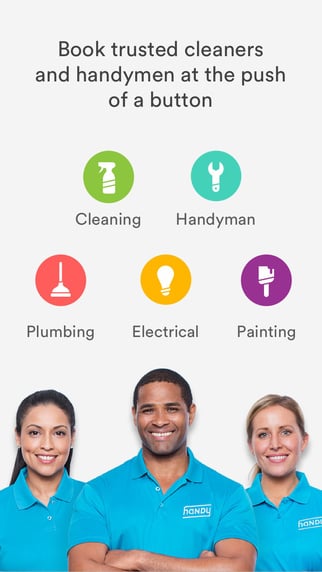The image features a rectangular banner with black text that reads, "Book Trusted Cleaners and Handyman at the Push of a Button." Surrounding this text are several colored circles, each representing a different service category: 

- A green circle with a spray bottle symbolizes cleaning services.
- A blue circle with a wrench signifies handyman services.
- A red circle with a plunger represents plumbing services.
- An orange circle with a light bulb denotes electrical services.
- A purple circle with a paintbrush stands for painting services.

At the bottom of the banner, there are three individuals, all dressed in blue collared shirts with white text. 

1. On the left is a woman with black hair, styled to reveal a dimple on her left cheek. She is smiling broadly, showing her teeth, and is wearing a shade of pink lipstick.
2. In the middle is a man also clad in a blue collared shirt. He is smiling and showing his teeth.
3. On the right is another woman, her hair pulled back into a ponytail. She is also smiling warmly.

The overall image conveys a trustworthy and professional team ready to offer a variety of home services.